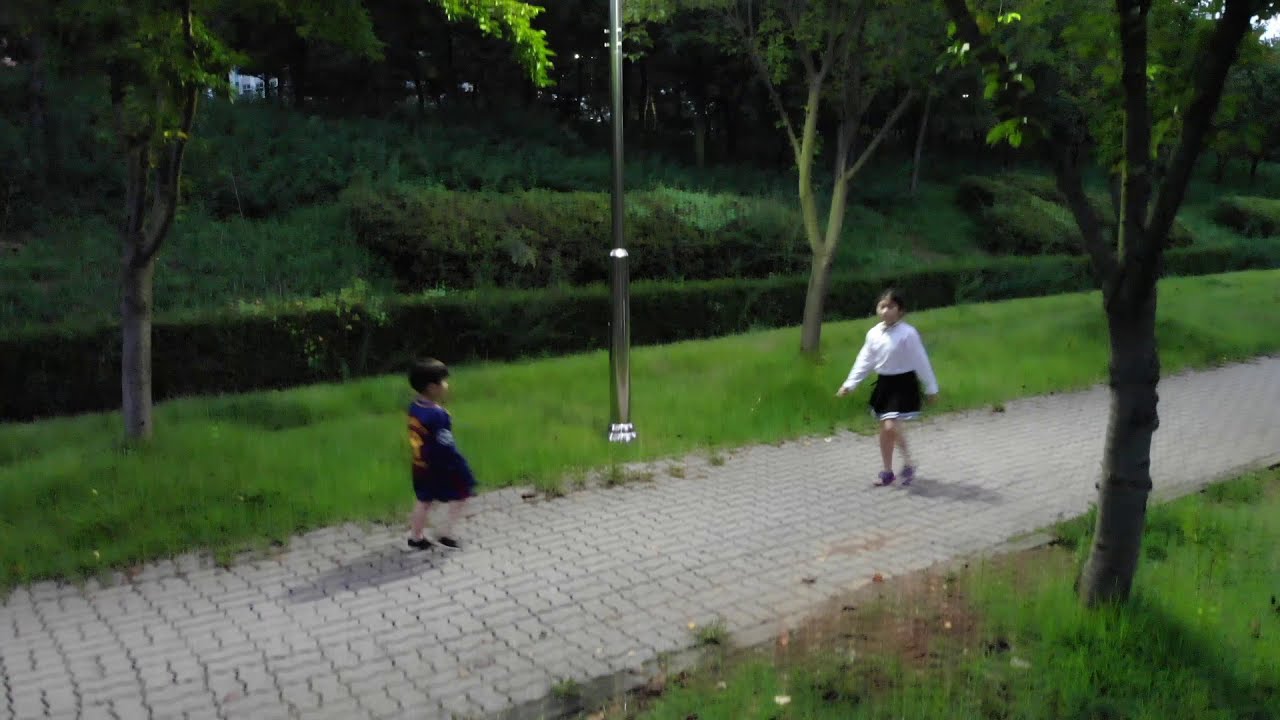In a picturesque, softly lit scene that resembles a painting, two young children meet on a brick-paved pathway in a park. The boy, positioned on the left, wears a dark blue jersey paired with black shorts and black tennis shoes. He has black hair and might have his hands in his pockets. The girl, to the right, is approximately six to eight years old and sports a long-sleeved white blouse, a blue sailor skirt with white trim, and sneakers. Her hair is pulled back into a low ponytail. They appear to be of East Asian descent and are slowly approaching each other. Between them stands a silver pole, likely a light post, shedding a gentle glow, suggesting it might be twilight or early evening. The pathway is flanked by lush green grass and sporadic trees, adding to the dreamlike quality of the image. In the background, a slope covered in bushes and trees rises gently, bordered by squared hedges that frame the path. The entire scene is enveloped in a serene and almost magical ambiance.